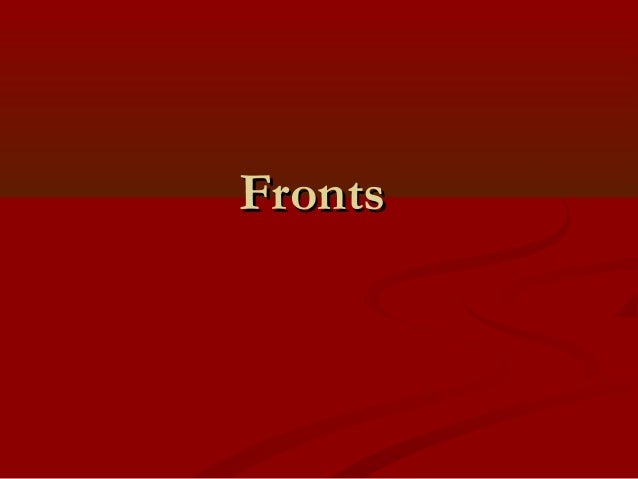The image depicts a horizontal rectangular PowerPoint slide with a two-toned red background. The top approximately 40% of the slide is a dark maroon or burgundy hue, slightly textured with horizontal grain that fades towards the top. The larger bottom section, roughly 60%, is a blood-red color, with faint, wavy dark red lines on the right side, resembling ripples on water. Where these two colors meet in the center, the word "FRONTS" is prominently displayed in off-white, bubble-like letters, with a slight black shadow. The "F" in "FRONTS" is capitalized, while the remaining letters are lowercase. This central text is the sole content of the slide.